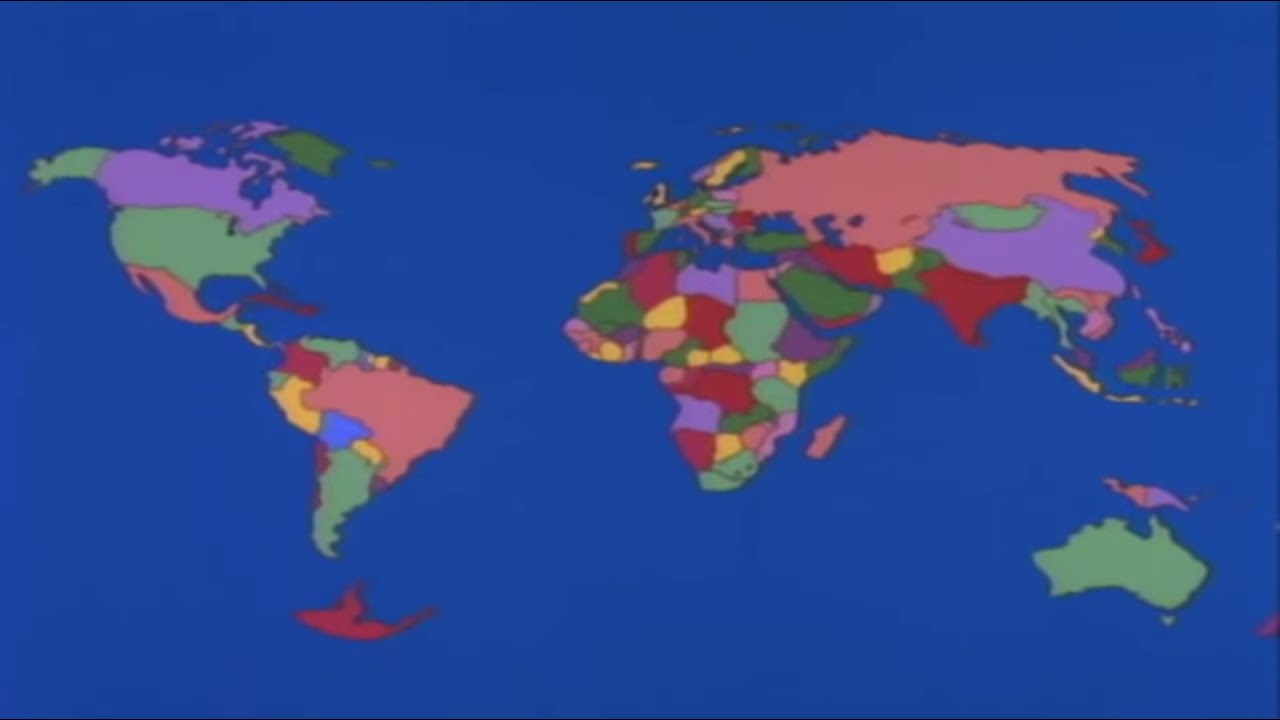This image depicts a flat digital map of the world, set against a royal blue background representing the oceans. The continents are vividly colored to distinguish different countries. On the upper left, North America is divided with Canada in purple, the United States in green, and Mexico in pink. Below lies South America, featuring countries in pink, blue, yellow, and red hues.

Prominently centered is Africa, displaying a rich palette of purple, red, yellow, blue, and green, while a distinctive blue area marks the Nile River. To Africa's top right, Europe and Asia are illustrated with countries in orange, green, purple, red, and blue, with Russia notable in a peach color and southern Asia in red. The islands of Japan stand out in green and purple.

In the bottom right corner, Australia is colored green, and New Zealand is depicted split between purple and pink. The map lacks any text, presenting a vibrant yet textless representation of the world. The image is somewhat blurry, but the colorful blocks clearly distinguish each country.